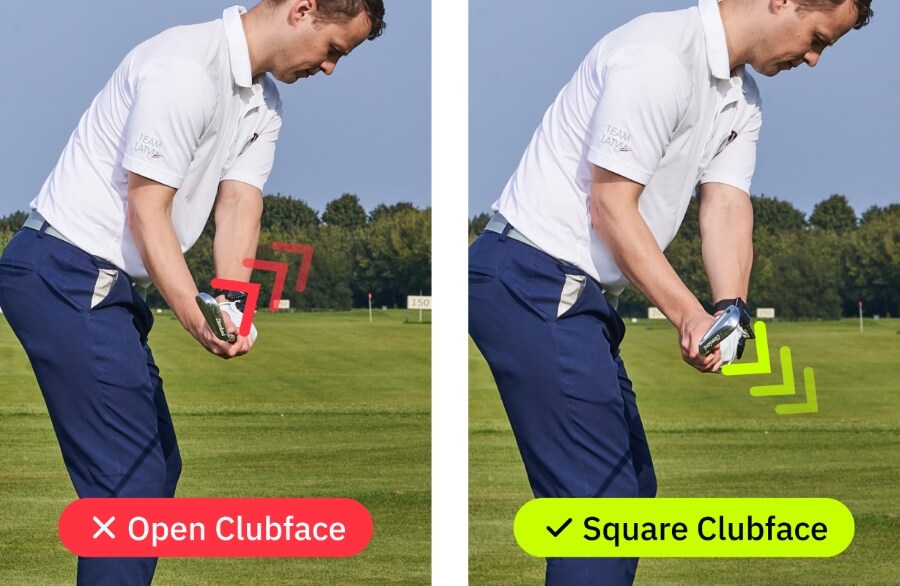The image features two side-by-side photographs of a golfer at the same moment in their swing, showcasing the orientation of the golf club face. The golfer is dressed in dark blue pants with a light blue belt, a white button-up polo with the collar unbuttoned, and is equipped with a white fingerless glove on their left hand and a black wristwatch. Behind the golfer, a serene golf course scene unfolds with verdant grass, distant flags, a line of trees, and a clear blue sky. 

In the left photograph, a red banner at the bottom reads "X, open clubface," depicting the golfer holding the club with the face pointed towards the top right corner. Red arrows emphasize the direction of the clubface. In the right photograph, a green banner at the bottom reads "✓, square clubface," showing the clubface oriented towards the bottom right. Green arrows highlight the new direction.